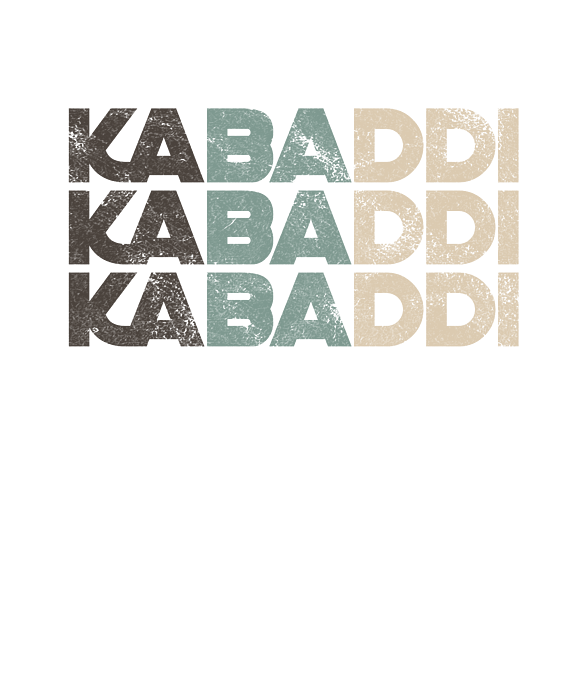The image is a horizontally-orientated text poster against a white background, featuring the word "KABADDI" repeated three times in capital letters. Each instance of "KABADDI" has a distinct visual style: the "K-A" is in bold black with visible streaks of white smudges; the "B-A" is a dark sky blue or aqua, displaying a slightly worn appearance with some paint missing; and the "D-D-I" is in a very light pink or beige hue, also showing signs of wear. Each repetition of the word is stacked one below the other, with no additional information or context provided within the image. The letters are block-styled, with the black "K" merging into the "A" slightly, while the other letters stand more isolated from one another.